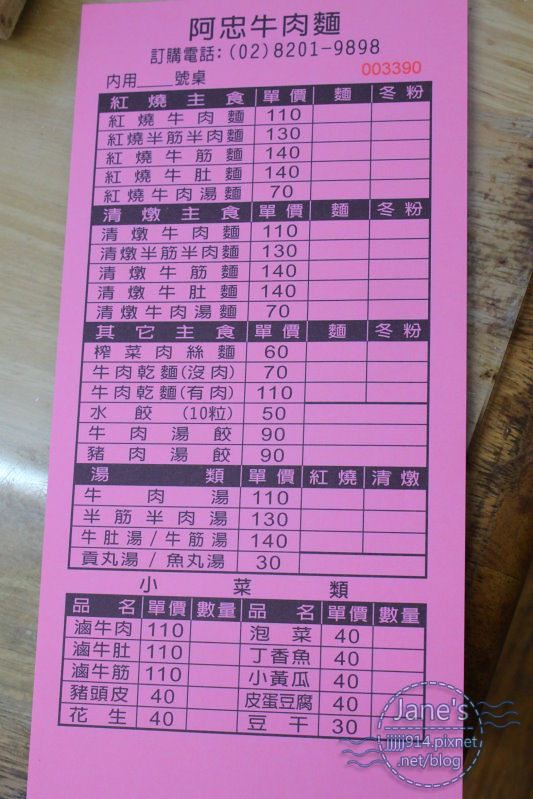This image depicts a vertically oriented, purple Chinese ticket or receipt placed on a brown wooden surface, likely a table or counter. The background enhances the prominence of the ticket, which features distinctive Asian characters and various numbers. At the top center of the purple ticket is a horizontal row of Chinese characters, followed by a series of mixed letters and numbers "028201-9898," which appear to be a phone number. Below this, additional text in Chinese, and numbers are arranged on the left, accompanied by corresponding prices or figures on the right. 

The ticket is divided into several vertical sections: the upper part consists of four blocks, each containing Chinese text with prices next to them—110, 130, 140, 140, and 70. A similar pattern of text and numbers (110, 130, 140, 140, and 70) continues in the subsequent blocks below. Towards the bottom, there is an additional block segregated into two halves, featuring Chinese text and numbers in one half, with blank spaces following the numbers. 

Additionally, a watermark on the bottom right corner indicates the origin of the image, reading "Jane's jjjjj914.pixnet.net/blog." The dominant colors and the structure of characters and numbers suggest that this could be a receipt or a score card often used in Chinese restaurants or establishments.